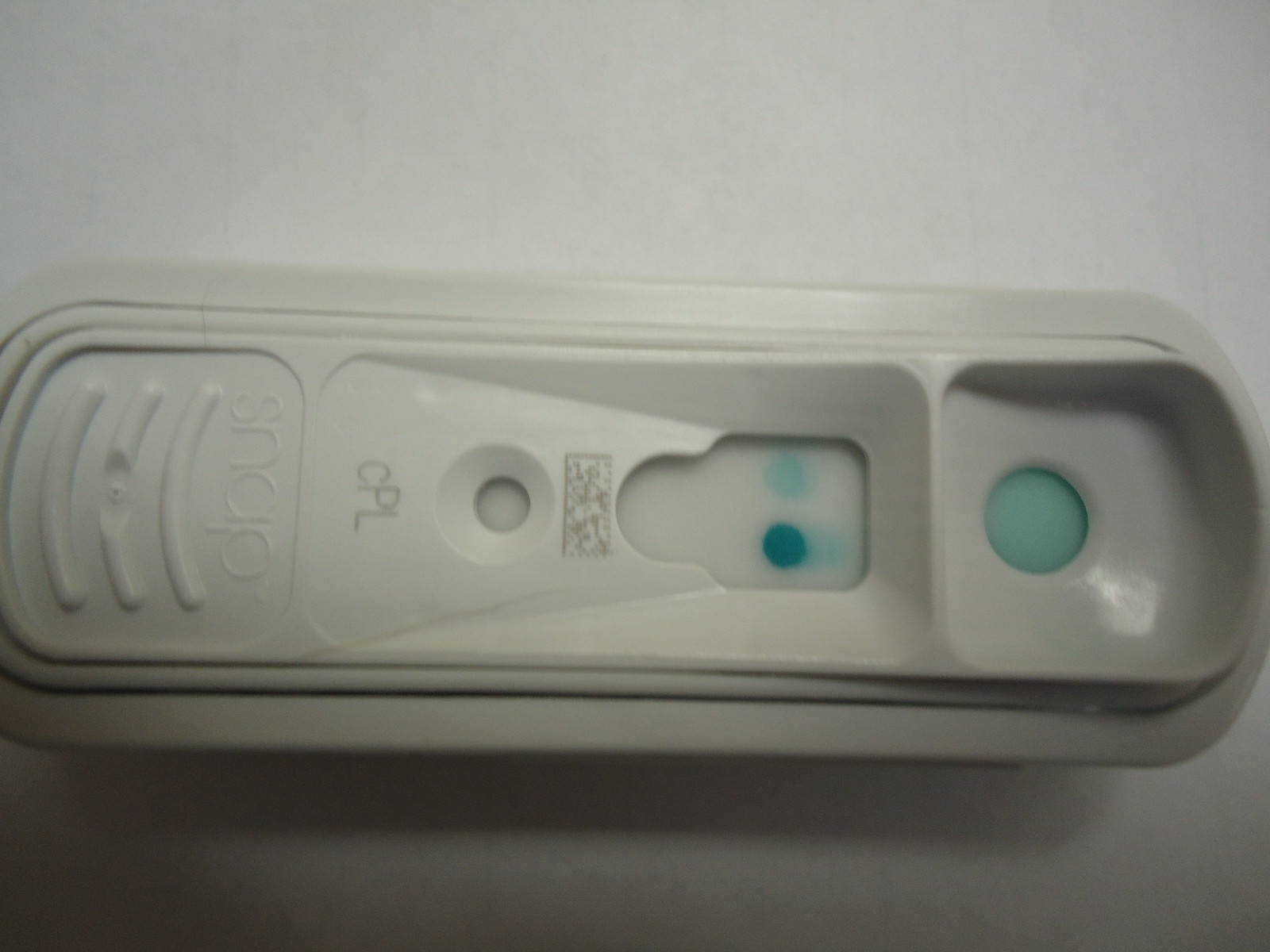The photograph features a rectangular, somewhat flimsy piece of white plastic that appears gray in the image. This object resembles a test result indicator, possibly for a pregnancy test. The plastic piece has gently curved edges. On the left side, there are three slightly upward curved lines, above which is the word "SNAP."

Further to the right, there is a section labeled "CPL," which features an intricate design: a circle with a smaller circle inside it, possibly for dispensing or some other function. Adjacent to this circle is a rectangular area filled with small squiggles.

To the right of this setup is the main indicator section, consisting of a square with a rounded portion on its left side that includes a dark blue circle and a light blue circle. The dark blue circle also has some light blue extending horizontally to the right.

Finally, the right-most section is almost square with rounded corners, featuring a light circle filled with light blue.